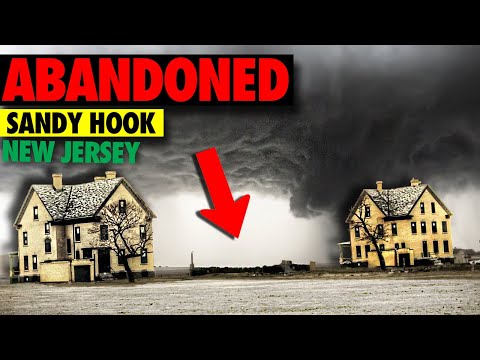The image appears to be a digital rendering or drawing depicting two identical, three-story homes, each adorned with large, slanted gray shingled roofs and multiple chimneys. They are positioned on either side of a vacant space that suggests a missing building, possibly due to damage from stormy weather. Dark, tornado-like grey clouds dominate the sky, creating a foreboding atmosphere. At the upper left corner, bold text in black and red within a black bar reads "ABANDONED" in red caps, followed by "Sandy Hook" in black within a yellow bar, and "New Jersey" in green within a green bar. A large red arrow points to the gap between the two houses, indicating the location of the obliterated structure. The image might serve as a dramatic thumbnail for a YouTube video.